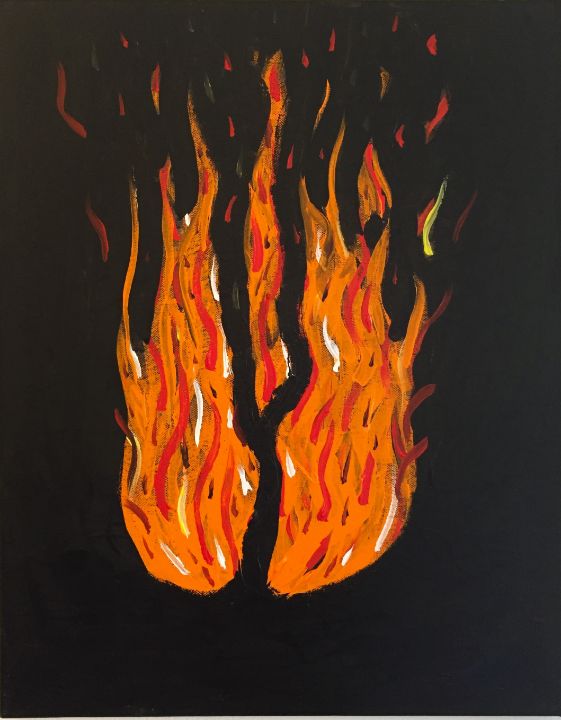This image showcases a painting of a flame set against a stark black background. The flame, composed of vibrant hues of orange, red, dark red, white, and a touch of yellow, stands prominently in the center. The fire is artistically split into three sections: one on the left, one on the right, and a central flame rising upwards, creating a dynamic and symmetrical composition. The style of the painting appears somewhat simplistic and crude, with broad strokes and minimal detailing. There is no text accompanying the artwork, focusing the viewer’s attention solely on the vivid depiction of the flame against the empty black backdrop.